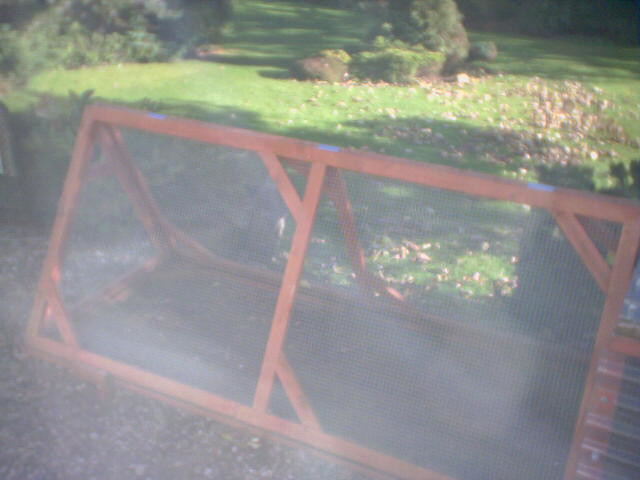The photograph captures an outdoor scene with a hazy, filtered effect, possibly as if viewed through a screen or window. The ground is covered in small pebbles and stones, subtly scattered around. At the center of the image stands an orange, metal, triangle-shaped structure, encased in mesh screens on all sides. In the backdrop, a lush green lawn stretches out, bordered by hedges on the left side and towards the center. Scattered brown leaves lie on the ground, adding a touch of autumnal ambiance to the scene.